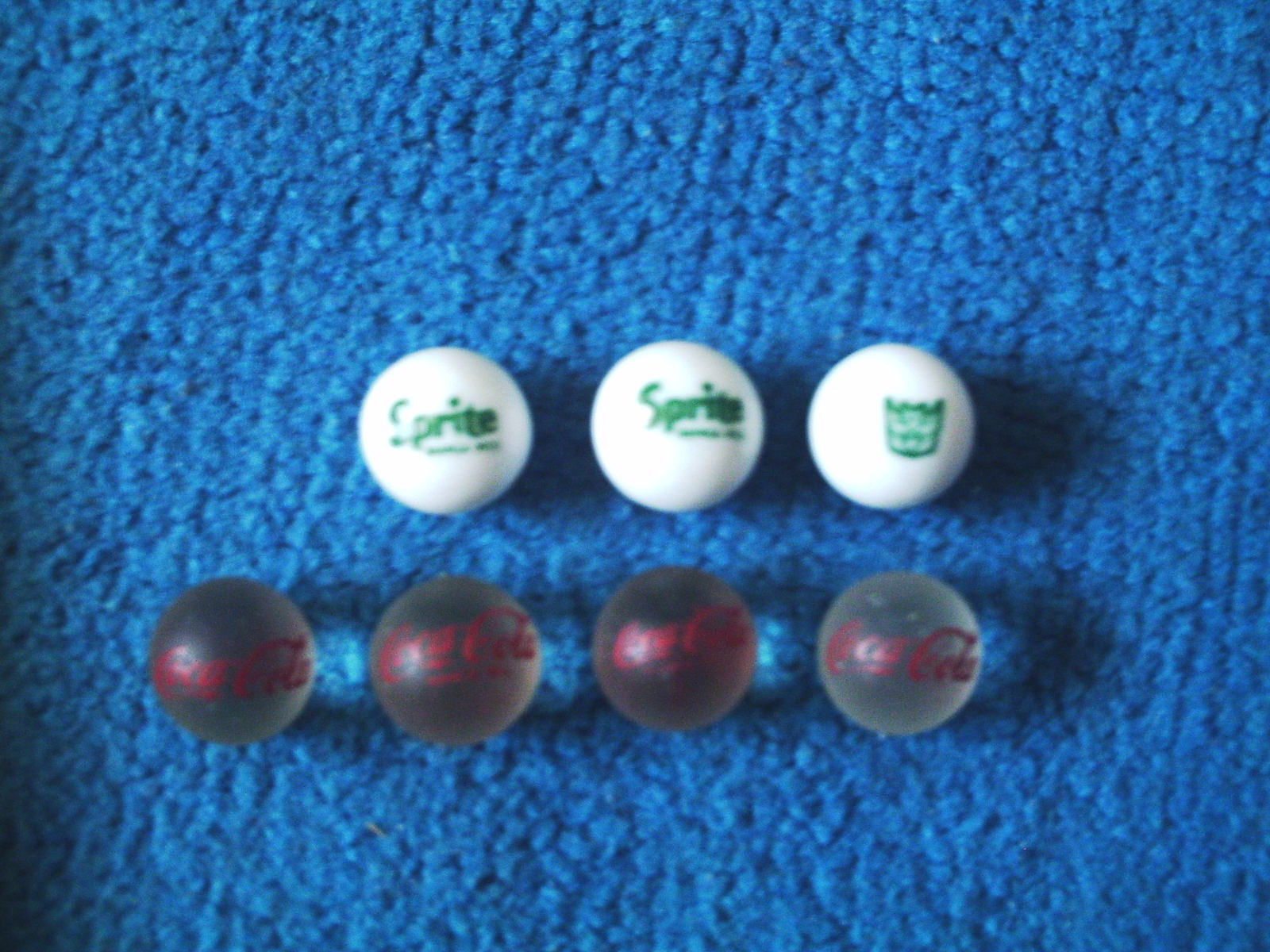A close-up photo taken on a light blue carpet, resembling the color of a blue sea, features seven marbles resting with their shadows cast to the right. The top three marbles are white, with two displaying the green Sprite logo, and the third on the far right showing a monstrous face, reminiscent of a Transformer villain. The four marbles at the bottom appear semi-transparent, giving off a murky clear look, and each is adorned with the Coca-Cola logo painted in red. The blue carpet beneath appears to shift from darker at the bottom to lighter towards the top, enhancing the contrast with the marbles.